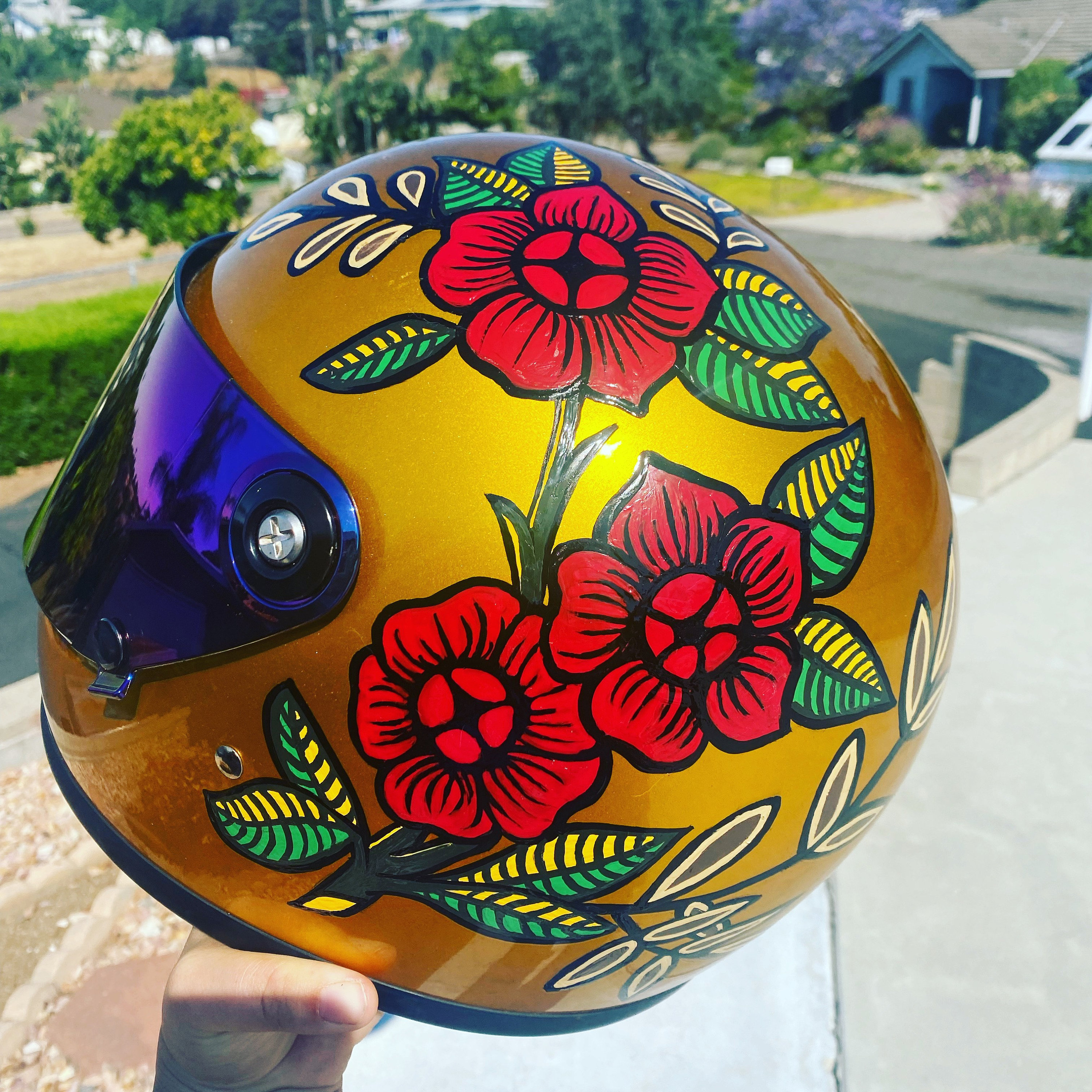In this outdoor daytime photograph, a person is holding up a strikingly customized motorcycle helmet. The helmet's base color is a lustrous gold, adorned with vibrant red flowers outlined in thick black borders. These floral designs, featuring delicate branches and a variety of leaves—green on one side and yellow or gray on the other—cover much of the helmet's surface. A dark-colored visor is fitted at the front, enhancing the practical yet artistic appeal of the helmet. The hand holding the helmet emerges from the lower left side of the image, partially obscured by what appears to be a rock, adding a touch of visual intrigue. The scene unfolds on a suburban sidewalk, with concrete and bricks visible on the lower right. In the background, houses with dark gray roofs and lush green trees are set against a backdrop of green grass, suggesting a serene neighborhood setting.